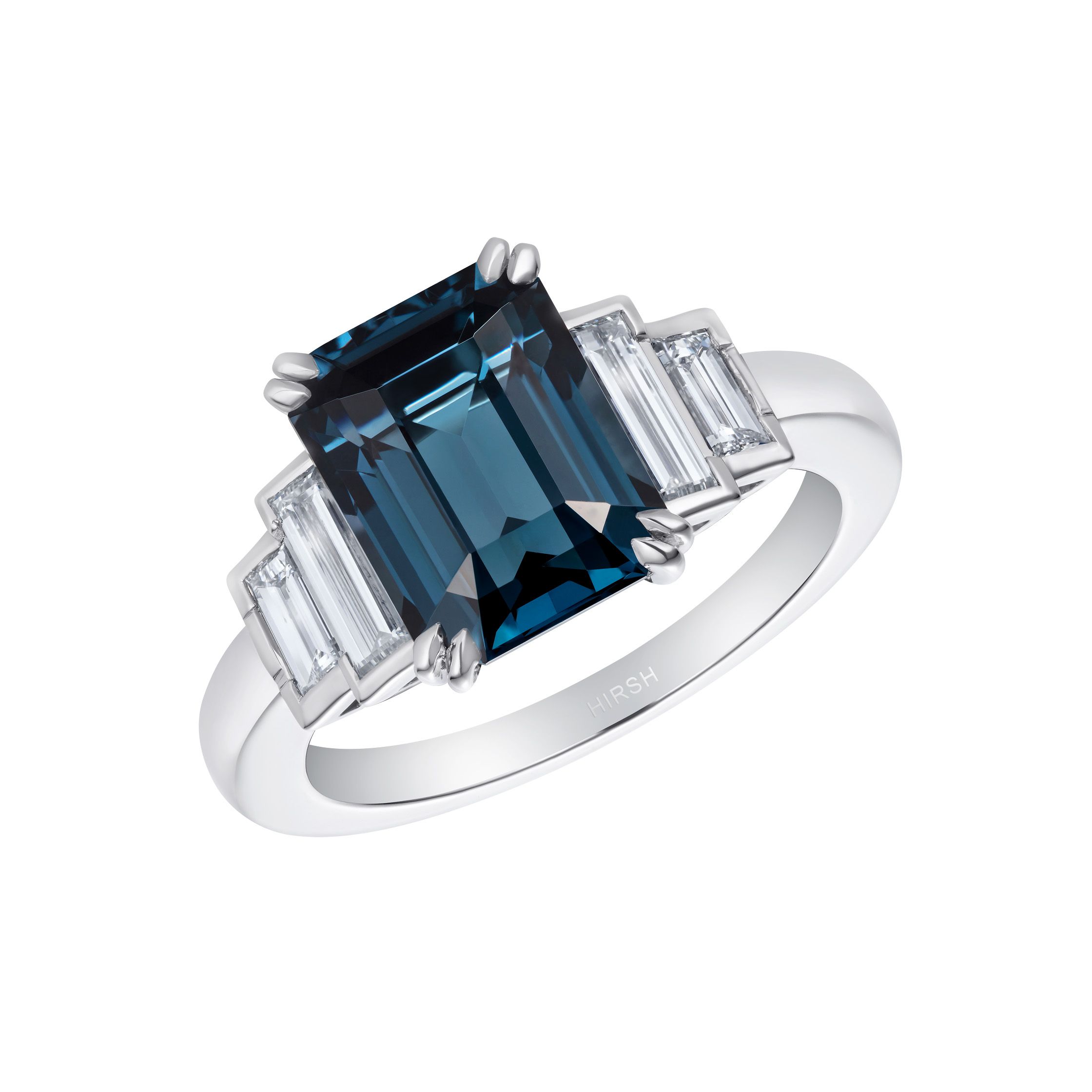The image showcases a stunning engagement ring made of silver, possibly platinum or white gold. The centerpiece of the ring is a large, square-cut blue sapphire—or possibly a blue topaz—secured by elegant silver prongs at each of its four corners. On either side of this central stone are pairs of baguette-cut white crystal plates or diamonds, with the ones closer to the sapphire being larger than those farther out. The exquisite craftsmanship is further accentuated by an engraving on the underside of the ring bearing the name "HIRSH" in lighter text. This intricate design makes it a truly gorgeous and eye-catching piece.